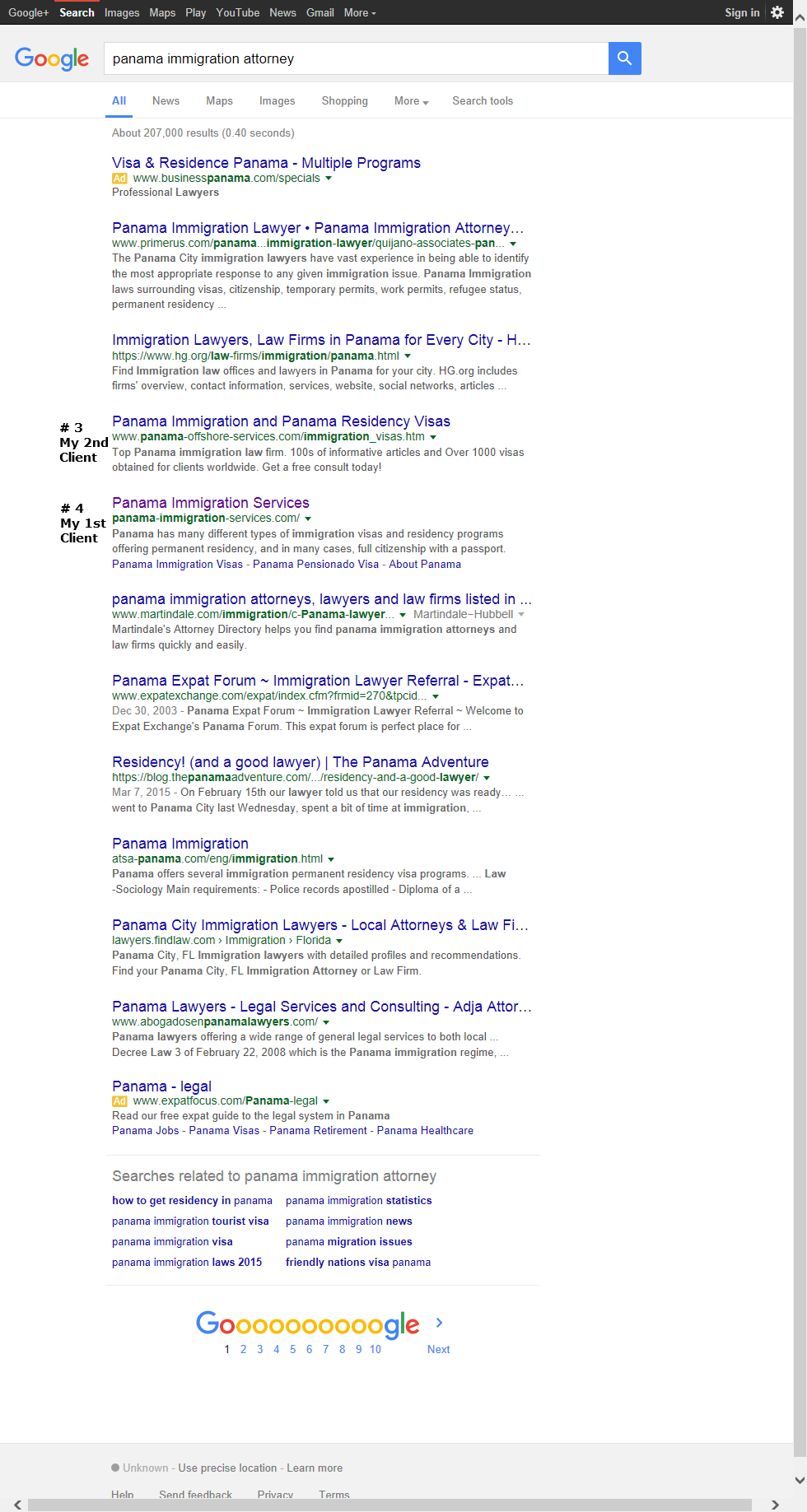A screenshot of Google search results for "Panama immigration attorney" is displayed. The top section includes a black navigation bar featuring options in white font: "Google," "Search," "Images," "Maps," "Play," "YouTube," "News," "Gmail," and "More." The upper-right corner shows a "Sign in" button and a gear icon. Just below, a gray bar houses the colorful Google logo and a search field containing the query "Panama immigration attorney," accompanied by a blue search button with a white magnifying glass icon.

Beneath this bar, the search results page offers several filtering options: "All," "News," "Maps," "Images," "Shopping," "More," and "Search tools." "All" is selected, and it displays approximately 207,000 results found in 40 seconds.

The first visible result is labeled as an ad that mentions visa and residence services in Panama with multiple programs. Following this ad, the organic search results start with listings for Panama immigration lawyers and firms, including specific options like "Panama immigration lawyer," "Panama immigration attorney," and "Immigration lawyers, law firms in Panama for every city." One of these entries has been altered, showing a written annotation on the left that states "Number three my second client," which comes off as boastful. 

Further down, another result titled "Panama immigration services" has a similar handwritten note next to it, stating "Number four my first client." Additional listings continue below, reiterating options for Panama immigration attorneys.